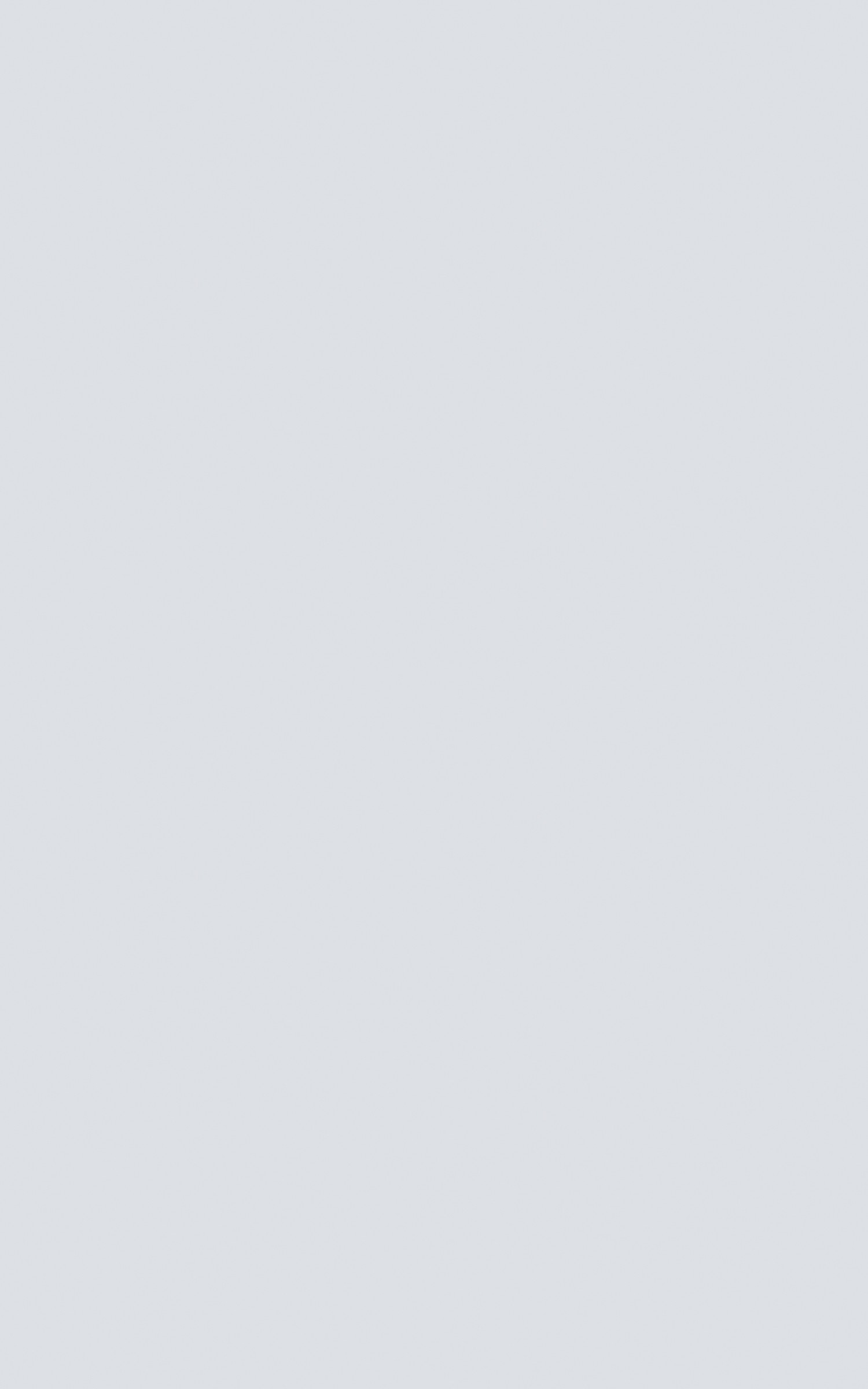The image depicts a simple, unadorned grey rectangle standing vertically on one of its shorter sides. The rectangle has a smooth, blank surface with no visible signs, symbols, letters, shapes, or images, making it a clean slate devoid of any distinguishing features. Its length is oriented along the left and right edges, while its width spans the top and bottom, with the length being notably greater than the width. The overall composition is minimalistic, offering no additional elements or context.